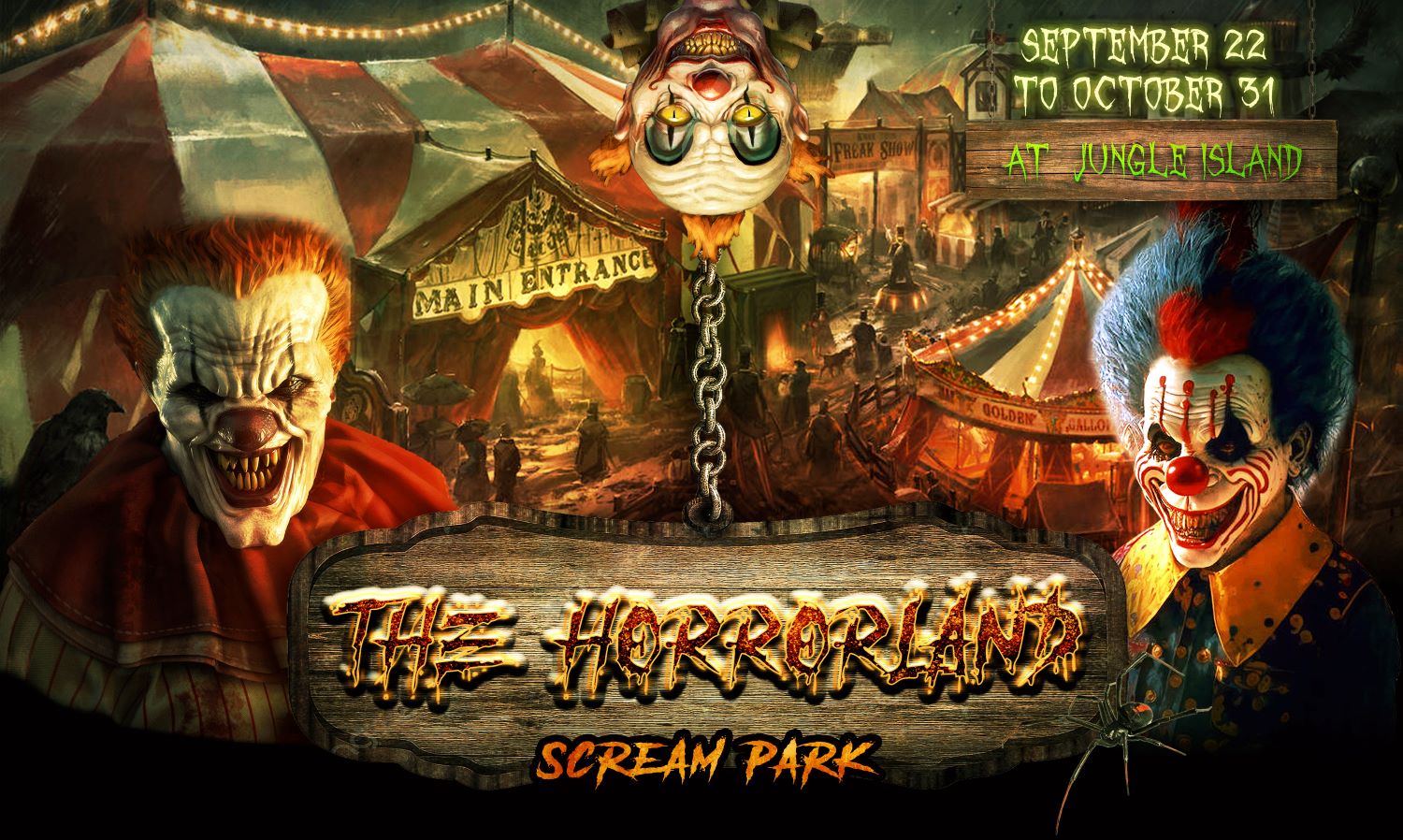This promotional artwork for "The Horror Land Scream Park" vividly captures the eerie essence of a Halloween-themed attraction. Dominating the bottom center is a 3D-rendered wooden plaque hanging by chains, inscribed with the text "The Horror Land Scream Park" in spooky red and yellow lettering. Flanking this sign are two menacing killer clowns: the one on the left with red hair and a chilling grin, and the one on the right featuring blue hair and makeup that resembles blood smeared across his face. Centrally placed above them, an upside-down clown with yellow eyes (but lacking the sharp teeth of the others) dangles from another chain.

In the upper right-hand corner, promotional dates are displayed in light yellow: "September 22 to October 31." Beneath this, text in green announces the location as "Jungle Island." The illustration's background, which contrasts with the rendered clowns in the foreground, showcases vintage circus scenes, including a red-and-white-topped tent labeled "Main Entrance," a freak show display, a merry-go-round, and figures dressed in 1800s attire wandering among these attractions.

This artwork, blending both detailed 3D renders and nostalgic illustrations, effectively conveys the spine-chilling allure of "The Horror Land Scream Park."